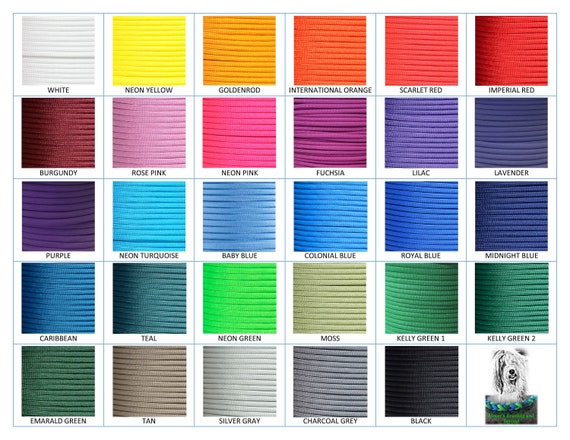In the image, there are six columns and five rows of different-colored squares, resembling paint swatches but with a rope-like, textured appearance, possibly indicating yarn or string. Each square displays a distinct color, with horizontal striations visible across each one. Starting from the top left and moving right, the colors are white, neon yellow, goldenrod, international orange, scarlet red, and imperial red in the first row. The second row includes burgundy, rose pink, neon pink, fuchsia, lilac, and lavender. The third row features purple, neon turquoise, baby blue, colonial blue, royal blue, and midnight blue. In the fourth row, the colors are Caribbean, teal, neon green, moss, kelly green one, and kelly green two. The final row consists of emerald green, tan, silver gray, charcoal gray, and black. Notably, the bottom right square diverges from the pattern, containing an image of a white fluffy dog's face with some green lettering that is difficult to decipher due to the image's small and compressed nature.